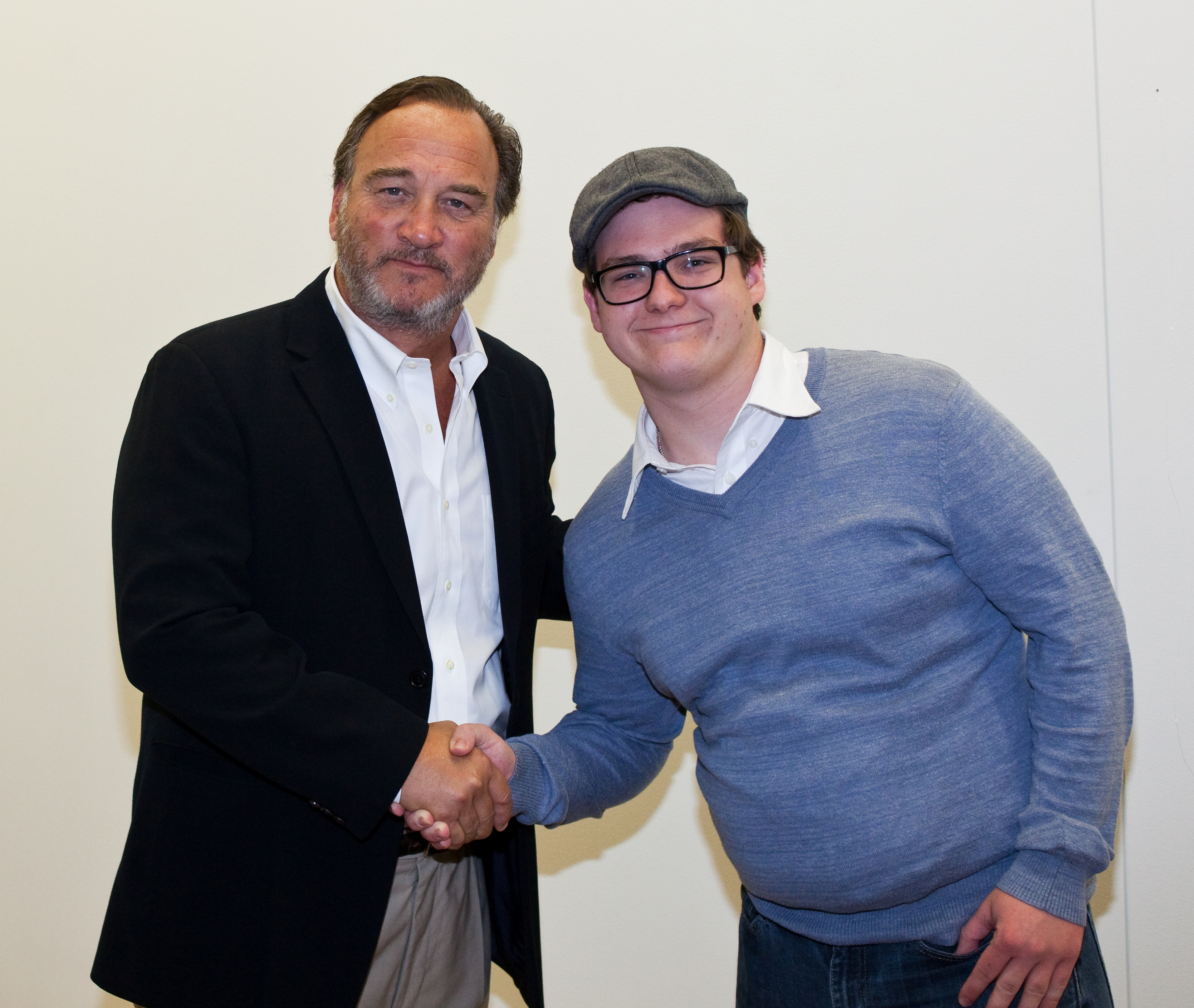This landscape-oriented color photograph captures a candid moment between actor John Belushi and an admirer. Both men are depicted standing against a cream-colored wall, shaking hands and gazing into the camera with subtle, half-smiles. John Belushi, positioned on the left, is distinguishable with his receding dark hair, graying beard and mustache. He's dressed in a white collared shirt left unbuttoned at the top, a black blazer, and khaki gray pants. He places his left hand supportively on the back of the man to his right. The admirer, leaning slightly towards Belushi, is attired in a blue v-neck sweater layered over a white collared shirt, a wool cap, dark-framed glasses, and blue jeans. Notably, his left hand casually sits near his pocket with his thumb tucked in. The style of the photograph is realistic and representational, highlighting the genuine interaction between the two.